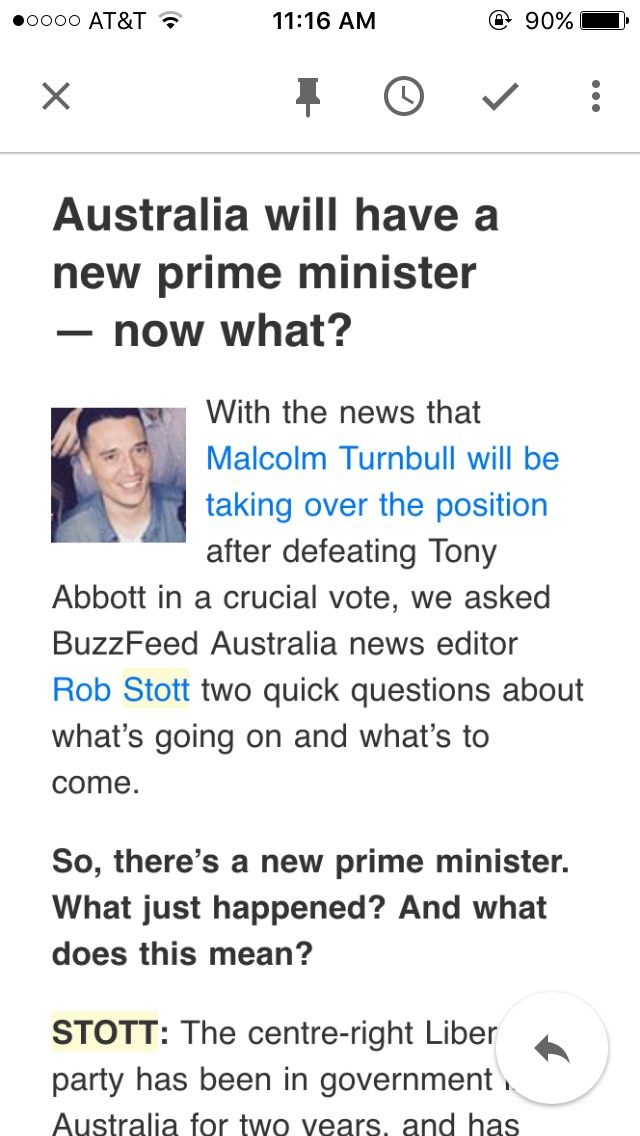The image details various indicators and text on a mobile device screen. In the top left corner, the network signal bar displays 1 out of 5 bars, indicating poor mobile network reception from the provider AT&T. The Wi-Fi signal icon, beside it, shows 2 out of 3 bars, suggesting moderate Wi-Fi connectivity. The device’s clock reads 11:16 AM. 

The main content of the image includes a news headline and article text, which states: "Australia will have a new Prime Minister now, or what?" The news highlights Malcolm Turnbull's victory over Tony Abbott in a crucial vote, leading to Turnbull taking over the prime ministerial position. The text mentions an interview with Rob Stott, BuzzFeed's Australian news editor, posing key questions about the recent political shift: "So there's a new Prime Minister. What just happened? And what does that mean?" It then touches on the political context, noting that the centre-right Libertarian party has been in government in Australia for 2 years, but the sentence is cut off before providing further information.